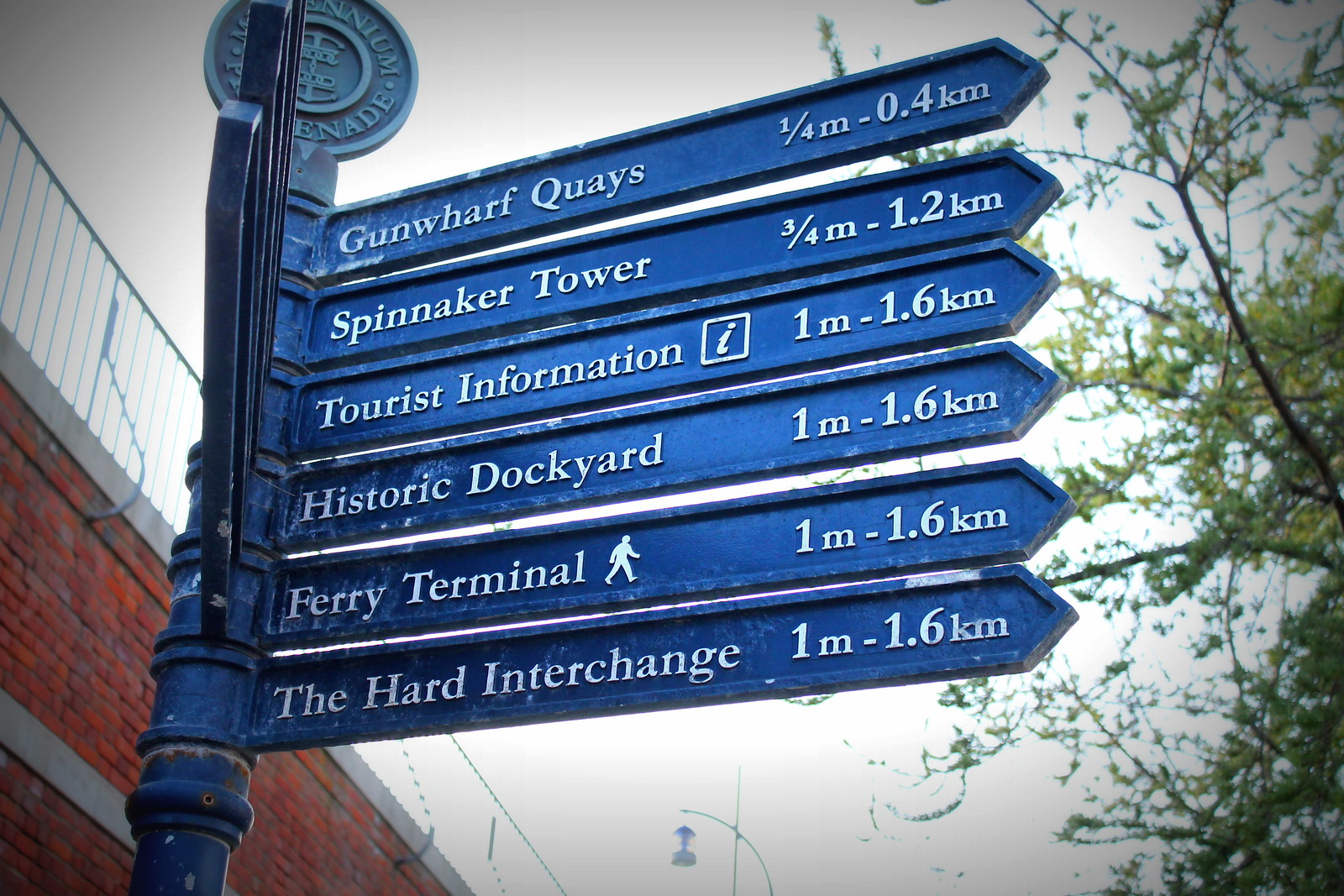In this image, an outdoor scene is captured in the middle of the day. Dominating the center of the composition is a tall, slender pole with a blue metal street sign pointing in various directions. The sign features six arrows with white text indicating directions and distances to key locations: Gunwharf Quays (0.25 miles / 0.4 kilometers), Spinnaker Tower (0.75 miles / 1.2 kilometers), Tourist Information (1 mile / 1.6 kilometers), Historic Dockyard (1 mile / 1.6 kilometers), Ferry Terminal (1 mile / 1.6 kilometers), and the Hard Interchange (1 mile / 1.6 kilometers). Notably, the sign for Tourist Information is marked with an 'i' symbol inside a box, and the Ferry Terminal sign includes an icon of a stick figure walking.

The photograph is taken from a low angle looking up into a bright, predominantly blue sky. On the left side of the image, a substantial brick bridge with a metal railing is visible, giving a hint of architectural interest, while on the right side, leafy branches of a tree extend into the frame, adding a touch of greenery. The color palette includes shades of blue, light blue, brown, gray, green, and tan, harmonizing natural and man-made elements in the scene.